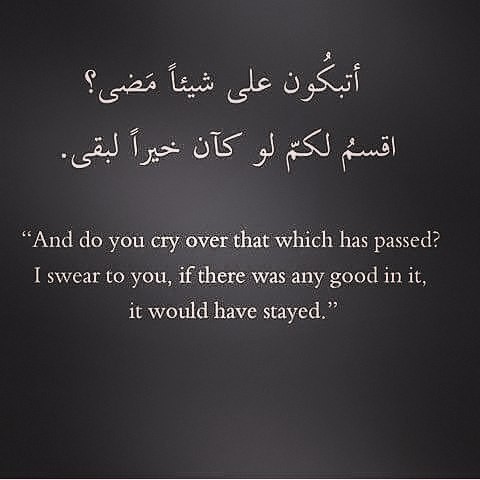The image features a near-square black background with subtle gray gradations towards the center. Presented in white serif font, it includes a quote in two languages. At the top, there are two lines of intricate, swirling Arabic script, presumably translating the English text below. The English quote, placed centrally, reads: "And do you cry over that which has passed? I swear to you, if there was any good in it, it would have stayed." Encased in quotation marks, this thought-provoking statement reflects on the futility of lamenting the past. The absence of additional images or colors ensures the focus remains on the powerful text.